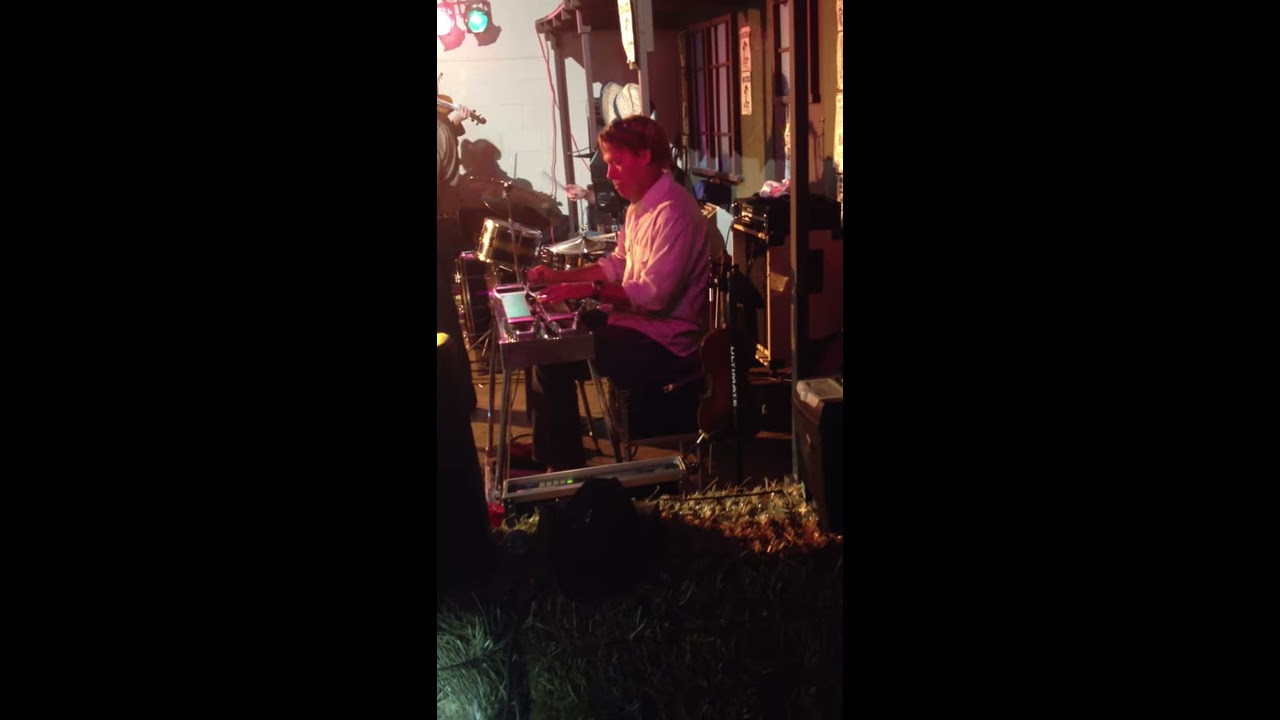In the center of the image, a male musician is absorbed in a performance, seated at a musical keyboard with a gray frame. He is distinguished by his white button-up shirt, black pants, and a black wristwatch on his left arm. His hands rest on the keyboard, immersed in playing. The performance takes place outdoors, evident from the building's front with windows behind him. The stage is demarcated by several hay bales stacked together in the forefront. The scene is dimly lit, with the only illumination coming from a green and red spotlight in the top left corner, casting a surreal pinkish hue on the man. To his left, there's a wooden violin on a stand, and a music mixer sits behind him. In the far distance, barely visible, another band member is poised at a black drum set, with only their arms and drumsticks discernible. The overall composition emphasizes the keyboard player's central role amidst a backdrop of musical paraphernalia, setting an atmospheric tone for the outdoor night performance.